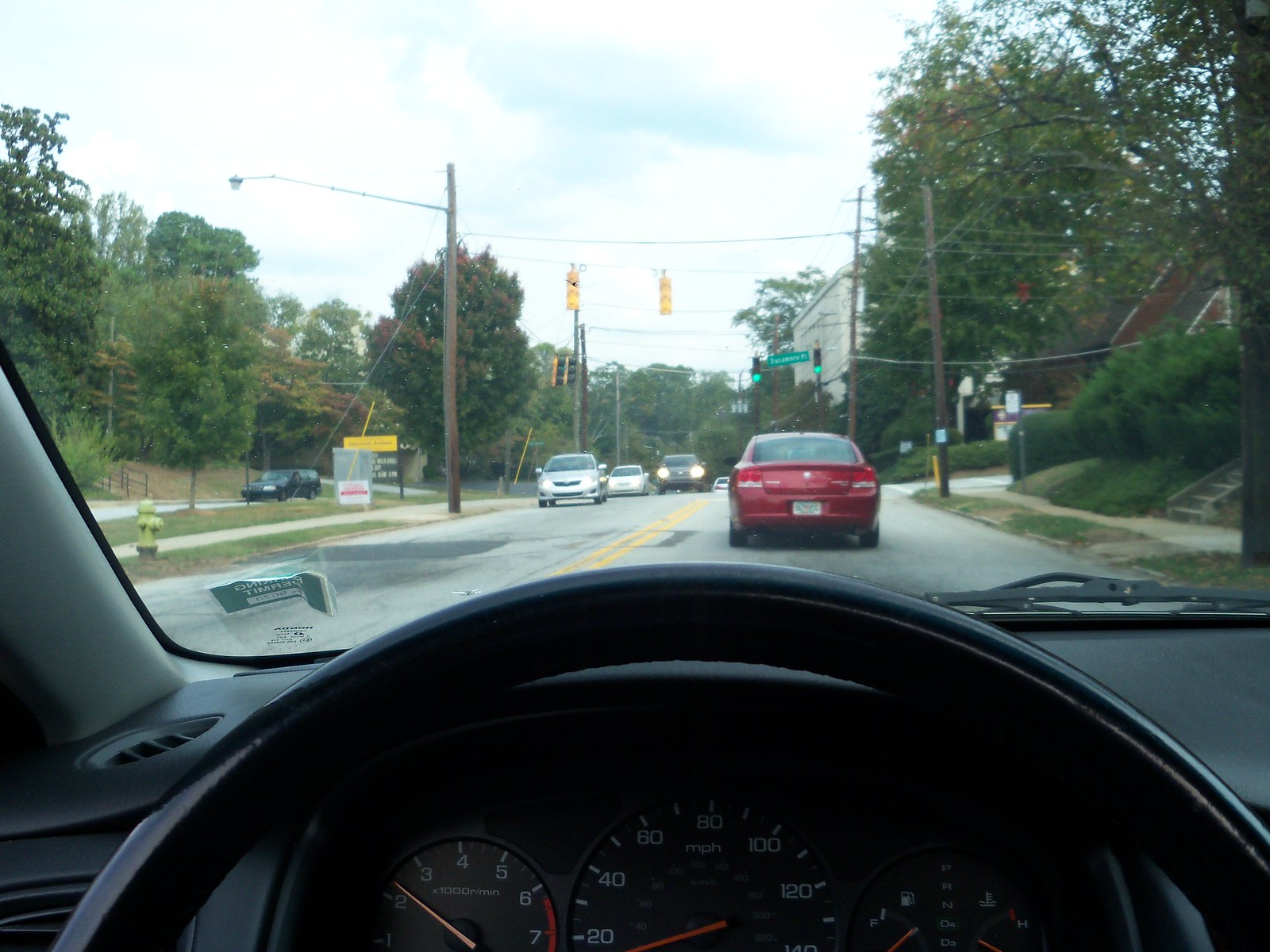The image captures a view from inside a car, with the steering wheel prominently positioned at the lower four-tenths of the frame. The dashboard is visible, displaying the odometer, speedometer, and other monitoring gauges. Through the windshield, the scene unfolds onto a vintage two-lane road with parked cars lining the sides. Overhead, telephone wires crisscross the sky, supporting traffic lights that dangle above an intersection. A red car is stopped at the light directly ahead. The background reveals a street sign, a building, and trees, suggesting a quaint, older neighborhood.